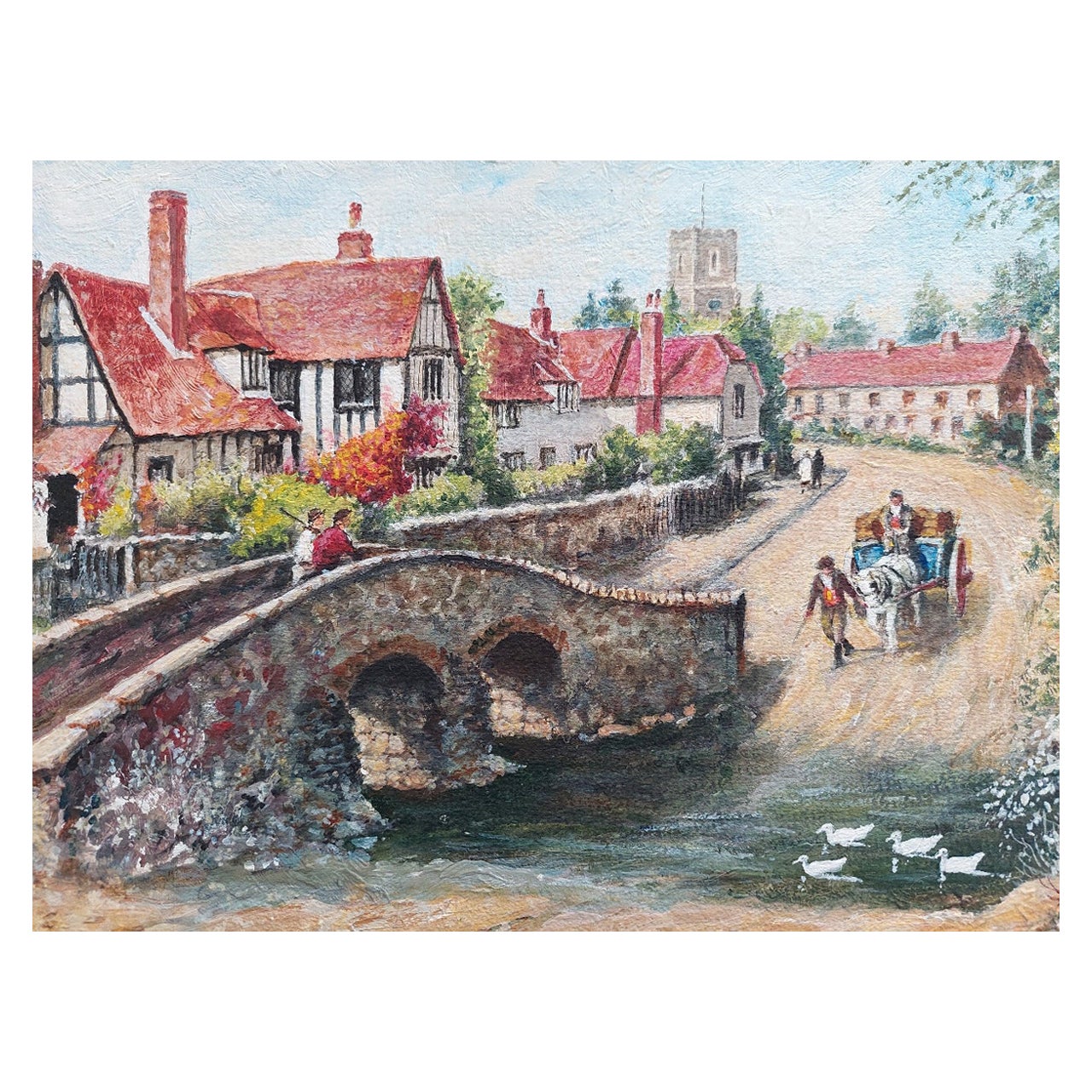This detailed painting depicts a rustic stone bridge crossing over a serene, dark green body of water, which is populated by four white swans swimming leisurely. Traversing the bridge from left to right, two figures stand out—one on the left dressed in a white top, and one on the right in a red top. In the background, more people are visible walking towards the bridge, one of whom is leading a white horse that is pulling a carriage occupied by a seated man. The bridge pathway and the surrounding area appear to be a light beige dirt road, adding to the quaint, old-time ambiance of the scene. The right side of the image features lush green tree leaves, and near the bottom, white flowers suggest the presence of flowering plants or trees. The sky above is mostly cloudy with patches of blue peeking through, enhancing the outdoor and historical feel of the artwork.